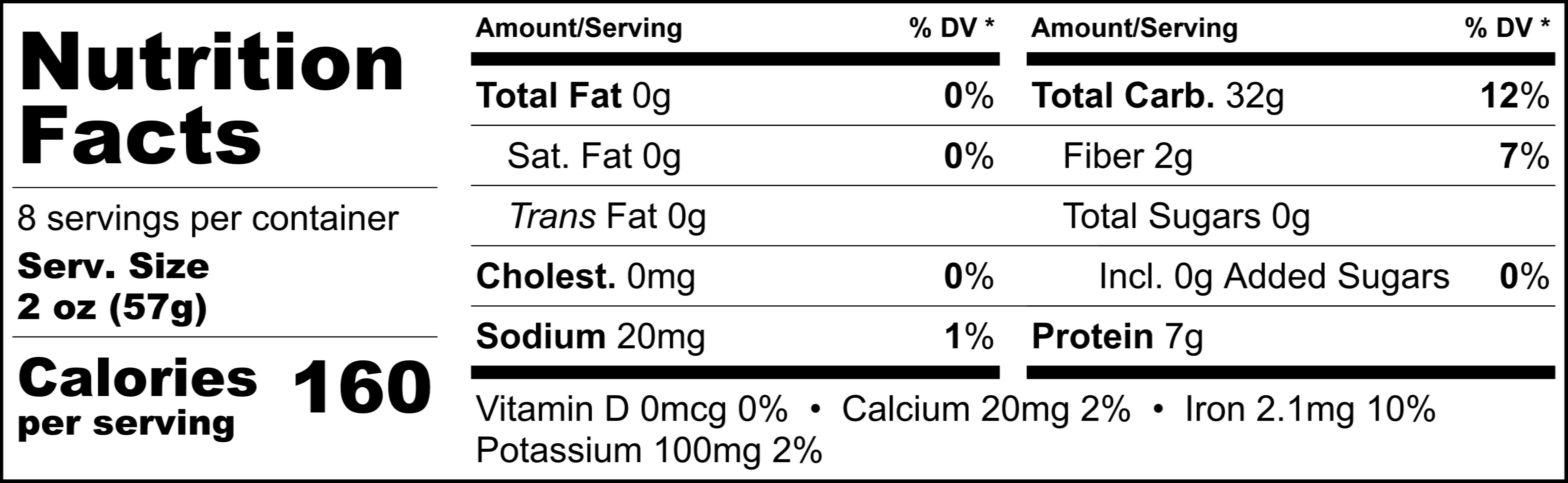This image showcases a detailed nutrition facts label typically found on the back of food product packaging. The label is displayed in a landscape orientation and has a rectangular shape. The entire background is white, while the text and borders are rendered in black for clear readability. 

In the top left corner, the label prominently features the title "Nutrition Facts" in bold letters. Directly below this, the label indicates that the package contains 8 servings, with each serving size being 2 ounces or 57 grams. Further down, also in bold, it states that each serving contains 160 calories.

The label is neatly organized into several categories, listing nutrient information and their corresponding daily values. These categories include:
- Total Fat
- Saturated Fat
- Trans Fat
- Cholesterol
- Sodium
- Total Carbohydrates
- Dietary Fiber
- Total Sugars (including added sugars)
- Protein

At the bottom of the label, additional nutritional information is provided for Vitamin D, Calcium, Iron, and Potassium.

While the label is comprehensive and detailed, the specific product it belongs to cannot be discerned from the label alone.